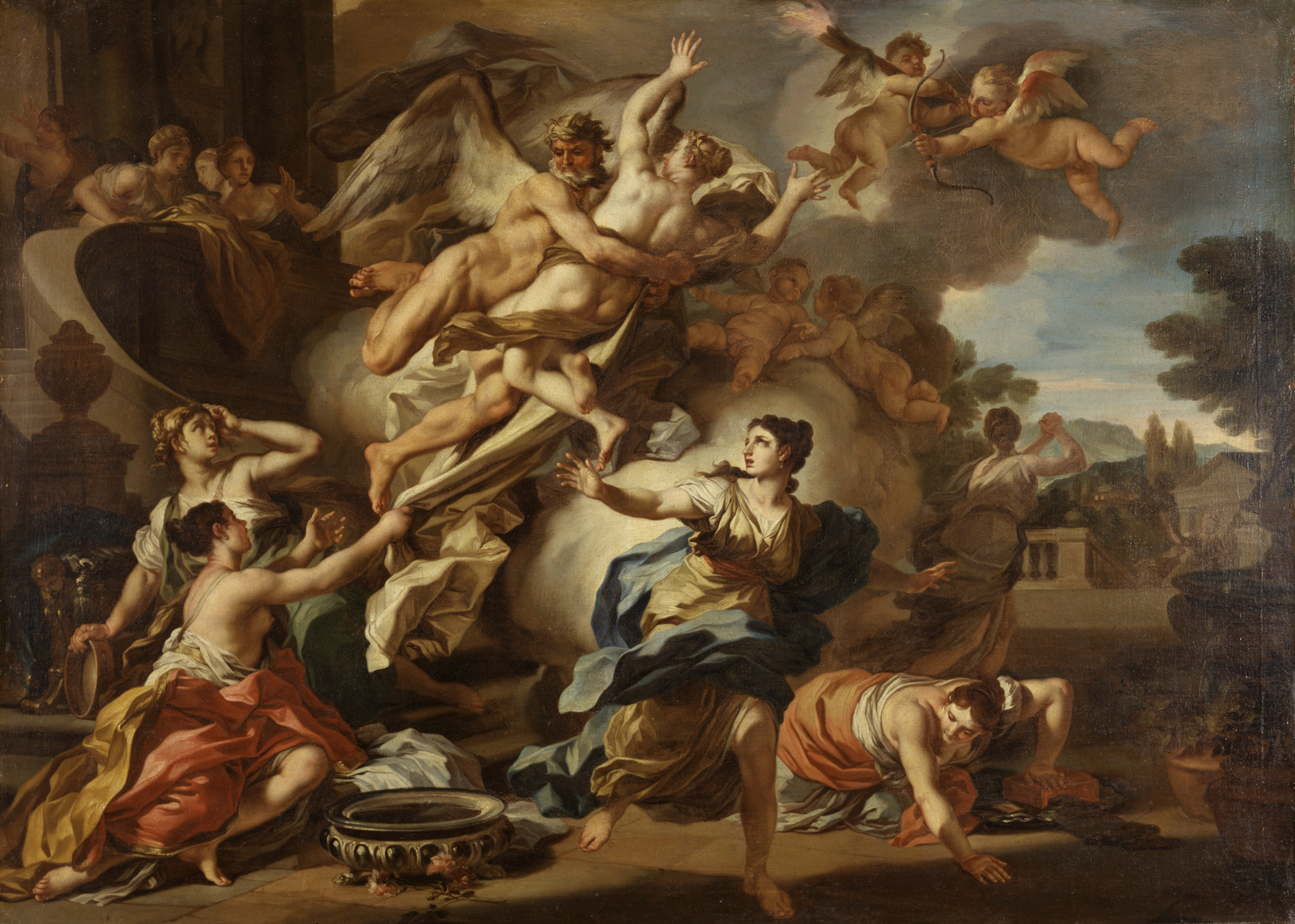In the foreground of this detailed oil painting, set against an overcast sky with hints of blue peeking through, four women are depicted on the ground amidst a scene of chaos and emotion. One woman appears to be fleeing while looking back, another is knocked over to the right, a third reaches up, grabbing a robe, and another looks up in shock and disbelief. All women are dressed in loose-fitting ancient-styled robes; the woman holding onto the robe has her chest exposed, perhaps symbolizing vulnerability.

Central to the painting, a dramatic encounter unfolds with a bearded angel, naked with large white wings, holding a woman he seems to be taking away. This interaction causes distress among the other women, with one on the ground clinging to the trailing fabric. Around them, winged cherubs, or cupid-like figures, add to the mythological theme, some with bows and arrows, others lounging on clouds.

In the background, behind a house, a tree is visible with a distant mountain rising majestically. Adding layers to the scene, a struggle unfolds; a winged man, possibly another angel, is seen hugging another figure, perhaps aiming to rescue or restrain. Women onlookers from a nearby palace balcony observe the unfolding drama, heightening the ancient, mythological ambiance of the painting.